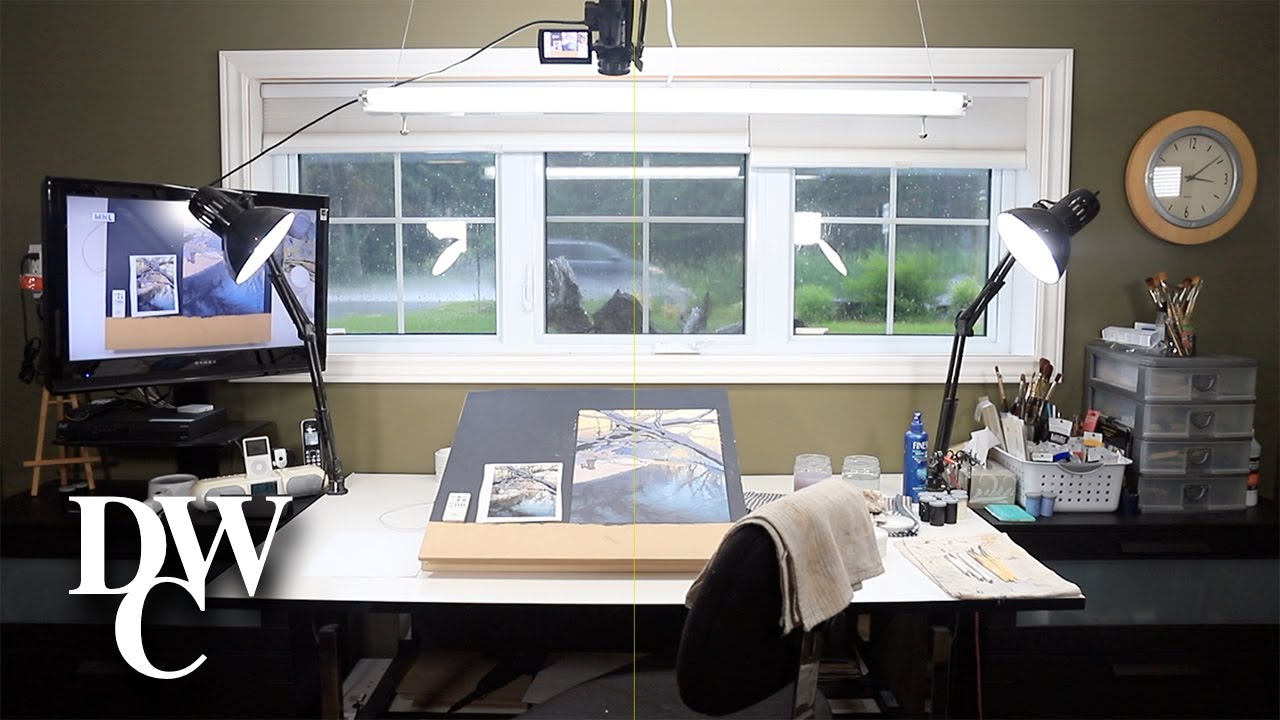This photograph showcases a detailed view of an artist’s home office, featuring a desk directly in front of a trio of paned windows. The desk is partially cluttered yet organized, presenting an artistic workspace with a painting in progress prominently displayed. Several gooseneck lamps, both black, illuminate the painting from the right and left sides, ensuring optimal lighting for the artist’s work. To the left of the painting area sits a black computer monitor. The desk is brimming with various art supplies, including multiple paintbrushes, pencils, and pens housed in different containers. 

Further, there are plastic drawers and containers for additional supplies. A chair with a towel draped over its back adds a personal touch, while a logo reading "DWC" is visible in the bottom left corner of the image. Above the workspace, affixed to a wooden round base on the back wall, is a gray clock showing the time as 3:08 p.m. Overhead, a bright fluorescent light fixture provides further illumination. In the background, you can glimpse a camera positioned at the top, pointing downwards, and an LED light. Lastly, the window reveals a rainy scene outside, adding a serene ambiance to the artist’s dedicated and creatively stimulating environment.